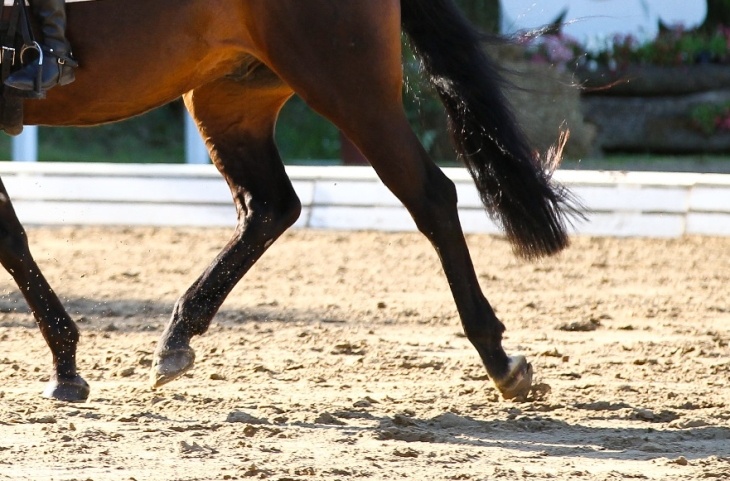The image captures the bottom right half of a chestnut-colored horse in motion, trotting leftward on light tan sand or dirt. Its legs and tail are black, and a small black leather boot, likely belonging to a rider, can be seen in the upper left corner, set in brown or black leather stirrups with silver clasps. The background features a blurry blue sky, green trees or bushes, and rocky formations in shades of tan and gray. There is also a white wooden fence with large horizontal planks, providing a clear boundary for this outdoor scene.